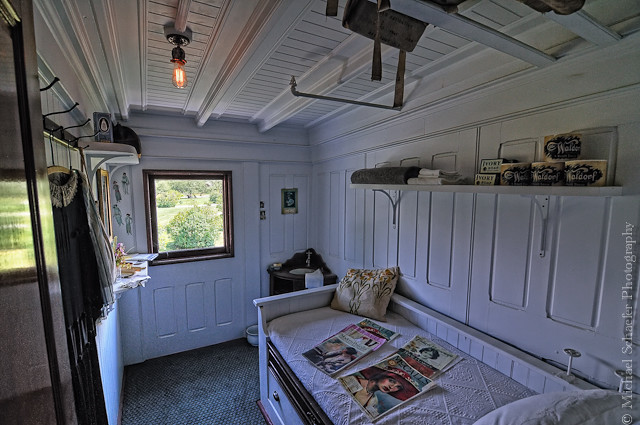The photograph captures an indoor room, presumably a small bedroom, with predominantly white painted walls and a white ceiling. The room, tidily arranged and well-lit, mixes natural and artificial light. On the left side, there is a closet door and a clothes rack or jacket hooks. A horizontally rectangular window, adorned with a picture frame, offers a bright view of green shrubs and a road outside. The floor is covered with a gray carpet, contrasting the white interior.

On the right side of the room, a child's daybed is positioned underneath a long shelf. The bed has a white sheet and is cluttered with a few magazines and a throw pillow. Below the bed, there's a drawer offering additional storage. Above the bed, the shelf holds several stacked containers, possibly cans, while a light fixture hangs from the ceiling, enhancing the cozy atmosphere. Overall, the room exhibits a clean, organized aesthetic with detailed elements of everyday living.